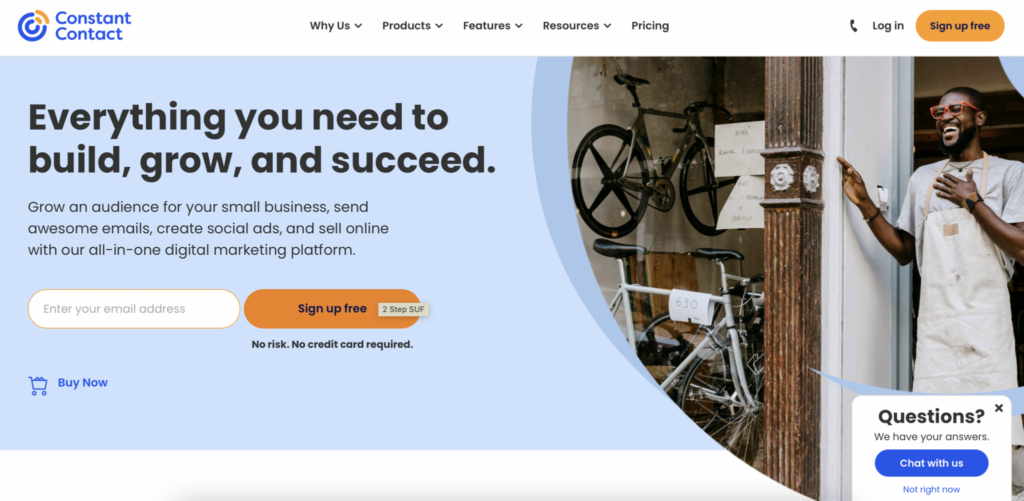### Caption:

This image captures a detailed screenshot of the Constant Contact business webpage. In the upper left-hand corner, the brand name and logo “Constant Contact” are displayed in blue. The top navigation bar includes the following labels from left to right: "Why Us?", "Products," "Features," and "Resources," each accompanied by a drop-down arrow, while "Pricing" stands alone without an arrow. 

To the right, icons for a telephone, "Log In," and "Sign Up Free" are visible. Dominating the central blue background, the black text reads, "Everything you need to build, grow, and succeed," followed by subtext outlining the platform's offerings: building an audience, sending emails, creating social ads, and selling online.

Just below, a white oval invites users to "Enter Your Email Address." Adjacent to it, an orange oval button reads "Sign Up Free." Below it is reassuring text, "No Risk, No Credit Card Required."

In the lower-left corner, there's a blue “Buy Now” button, while the right side features a vibrant image of an African-American man standing in a doorway, laughing with his left hand on his chest and his right hand on the wall. Bicycles are visible in the background, suggesting the setting might be a bicycle store or repair shop.

At the bottom right, a small white box offers customer assistance: "Questions, We Have Your Answers," with a blue oval button that reads "Chat With Us," next to an option that says "Not Right Now." This screen is clear and inviting, reflecting a user-friendly digital marketing platform.